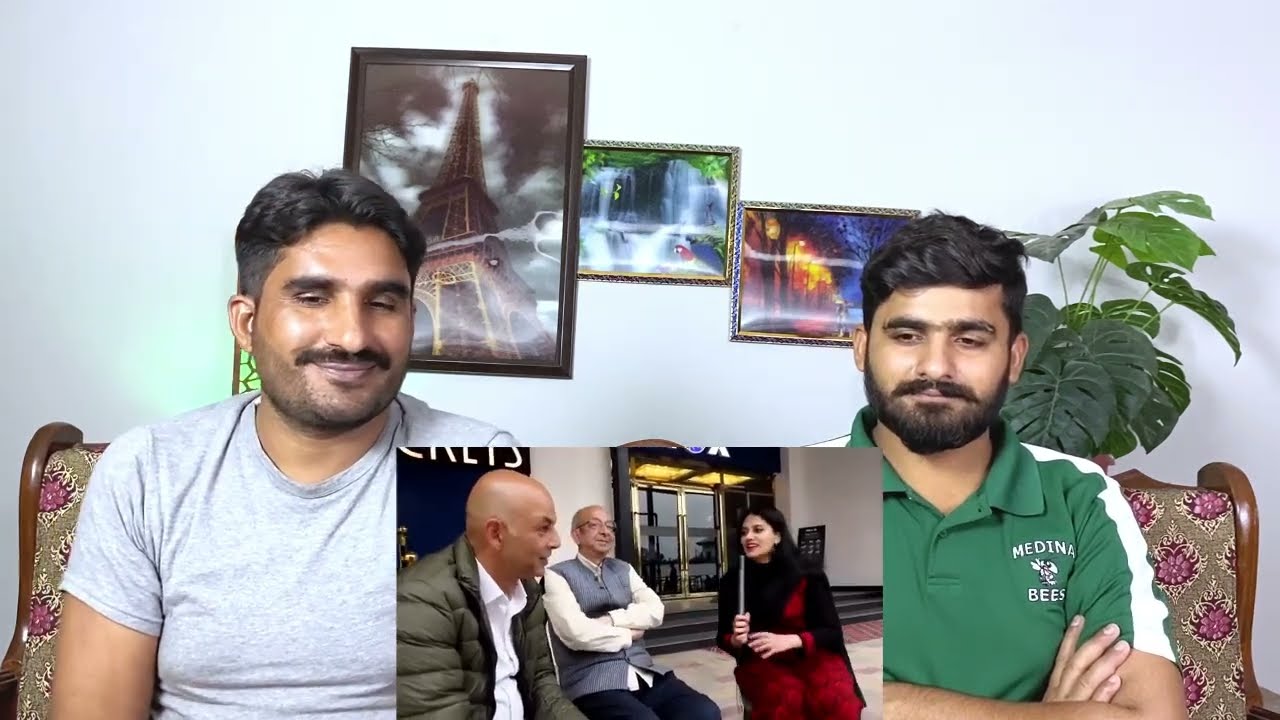In this image, which appears to be a still frame from a reaction video, two Middle Eastern men are seated on a wooden-framed couch with a brown and purple floral design. The man on the left is wearing a light gray short-sleeve t-shirt, has medium-length black hair, a five o'clock shadow, and a mustache. He is smiling and looking towards the center. The man on the right is dressed in a green polo shirt with white stripes on the sleeves, has medium-length black hair, a beard, and a mustache, and has his arms crossed while also gazing towards the center. 

In the bottom center of the image, there is a picture-in-picture thumbnail reminiscent of a reaction video setup, showing what they are watching. This inset features a Middle Eastern woman holding a microphone and interviewing two older Middle Eastern gentlemen. They are outside a building with glass doors, steps, and an overhang. Behind the two seated men reacting to the video, there is a large potted plant and three pictures on the wall, including one of the Eiffel Tower and another of waterfalls.